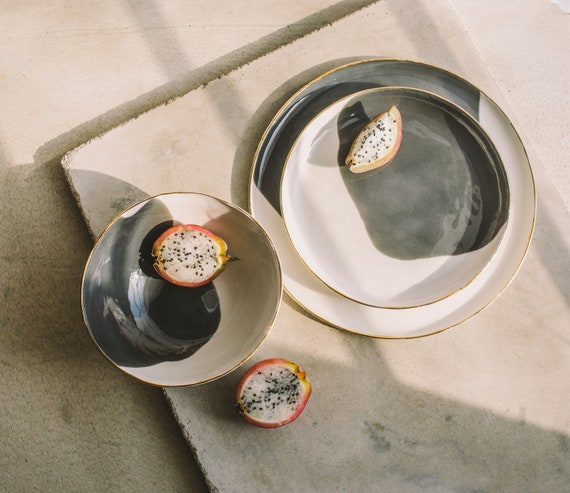In this landscape-oriented color photograph, we are looking down onto a light gray, almost white, textured surface, possibly a cloth or countertop, with visible little gray cracks. Positioned on this surface is an old, whitewashed wooden board placed at an angle from the top left to the bottom right. The edges of the board are beginning to crumble, adding a rustic charm to the composition.

On the right side of the board sits a large, circular ceramic plate with a smaller, shallow bowl inside it. Both the plate and bowl have a white center with a striking black blob, creating an abstract, yin-yang effect, and a thin gold rim around the edges. Inside the bowl is a quarter slice of dragon fruit, which has a vivid pink skin with a white interior speckled with small black seeds.

To the left of the setup is a matching bowl resting on the board. It holds three-quarters of a dragon fruit slice, similar in appearance to the one on the right. Below this bowl, lying directly on the board, is another slice of dragon fruit, showcasing the same pink skin, white flesh, and black seeds.

The photograph exudes a high level of detail that creates a sense of realism, making it hard to distinguish if it’s a photograph or a meticulously done painting. The arrangement of the dragon fruit pieces and the elegantly contrasting black and white ceramic dishes create a visually appealing, harmonious composition.